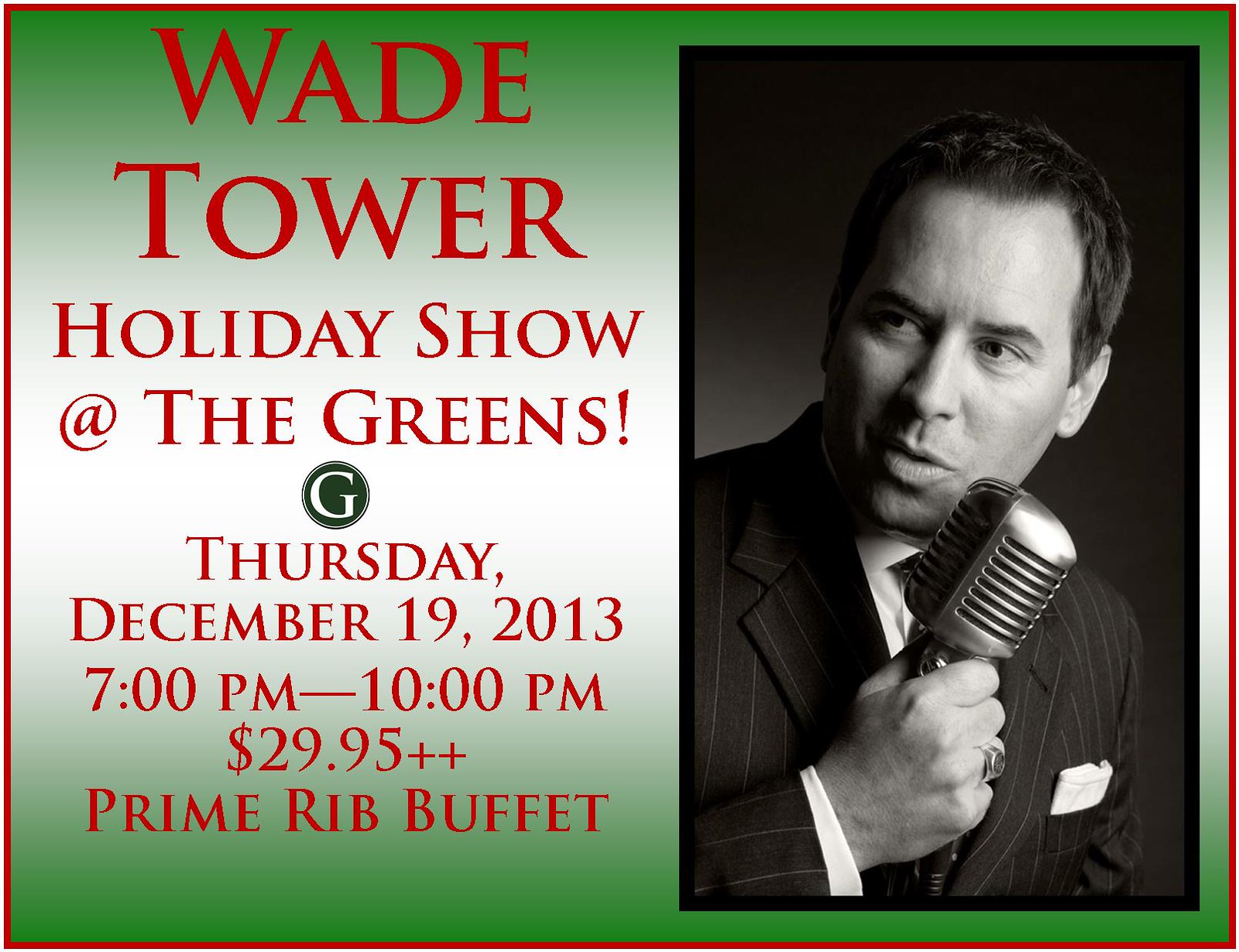The rectangular image, wider than it is tall, features a festive design with a thin red border encasing a green background that transitions to white in the middle. On the left half, in bold red print, the text reads "Wade Tower Holiday Show at the Greens." Below it, the details continue with "Thursday, December 19, 2013, 7:00 PM - 10:00 PM, $29.95, plus Prime Rib Buffet." Nestled between the event title and the date, there is a green circle with a white capital G. The right half of the image showcases a black-and-white portrait of a man with short hair, dressed in a gray pinstripe suit over a white button-up shirt, with a white handkerchief in his front pocket. He is depicted from the mid-chest up, bending slightly forward and looking to the left, while holding an old vintage-style microphone in his right hand, which also displays a ring. The man is in a moment that suggests he is singing into the shiny, round microphone.